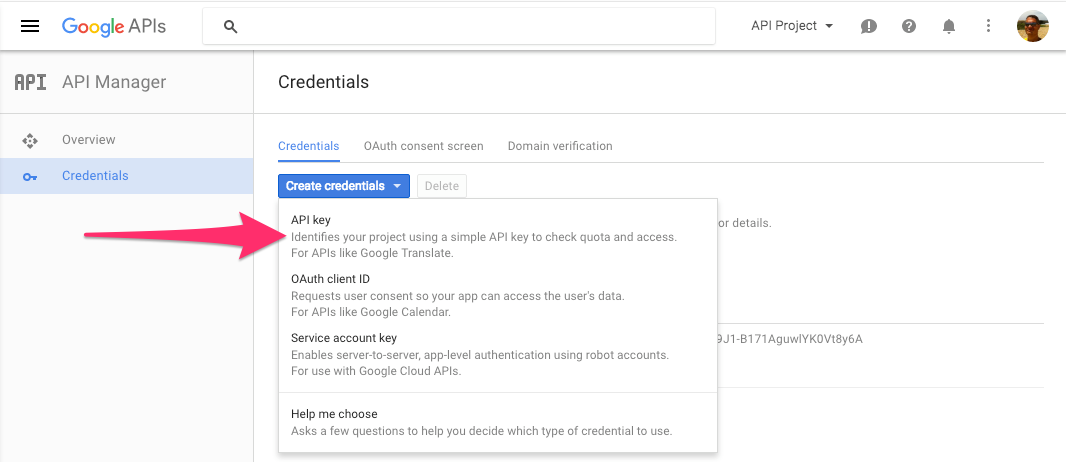The image appears to be a screenshot taken from a smartphone or smart device, with a horizontal orientation stretching from left to right. The top and left sides of the image are bordered by a thin gray line, while the bottom and right sides lack such borders.

At the very top left corner, there are three horizontal black bars, commonly signifying a menu or more options. To the right of these bars, the Google symbol appears, accompanied by a magnifying glass icon representing the search function. Adjacent to these, a white search bar is displayed. Moving further right, the text "API project" is visible, followed by several icons: an exclamation point within a circle, a question mark, a bell, three vertical dots (likely indicating additional options), and a profile picture within a circular frame.

On the left side of the screen, a gray sidebar contains the text "API, API Manager." Within this section, the options "Overview" and "Credentials" are available, with "Credentials" highlighted in blue, indicating it is the current selection. The word "Credentials" is displayed prominently against a white background.

Beneath this header, in blue and underlined, "Credentials" is again listed as the chosen tab. Below this is a series of options: "O, Authorization," "Consent Screen," "Domain Verification," "Create Credentials," and "Delete." Following these options, bold black text categorizes different types of credentials: "API Key," "OAuth Client ID," "Service Account Key," and "Help Me Choose," each accompanied by a brief description.

A red arrow points specifically to the "API Key," drawing attention to this particular credential option.